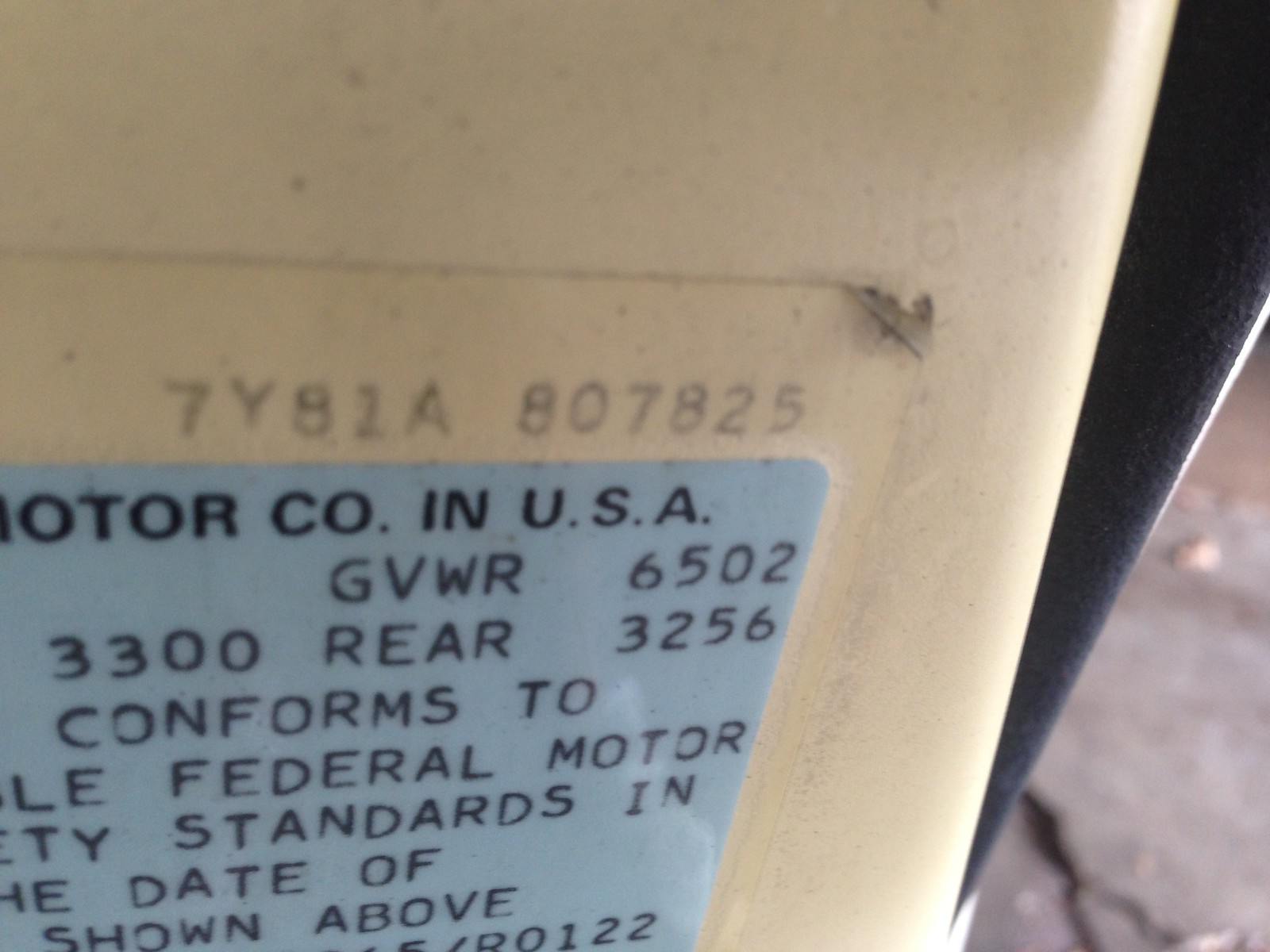The image is a close-up of a vehicle identification plate partially affixed to a tan-colored surface, possibly inside a car. The placard itself is light blue with black text, with some parts of the sticker starting to peel off, particularly the upper right corner. 

At the top of the visible text, the plate reads "7Y81A807825," albeit slightly out of focus. Below this number, against the blue background, it says "MOTOR COMPANY IN USA," partly obscured, likely denoting Ford Motor Company. Further details include the gross vehicle weight rating (GVWR) listed as "6502 lbs," with additional weights of "3300" and "3256" for different sections of the vehicle. 

The text continues with "conforms to LE federal motor," followed by fragmented words "TY standards in," and "HE date of," indicating compliance with federal motor standards and a date specification. There is also a partial tire size inscription that reads something like "R0122."

The sticker appears to be affixed near what might be a black tube, adding to the intricate details. The background appears to show some additional elements like a metallic beige panel, possibly part of the car's interior or another component. Overall, the colors in the image include light blue, tan, black, and a hint of gray.